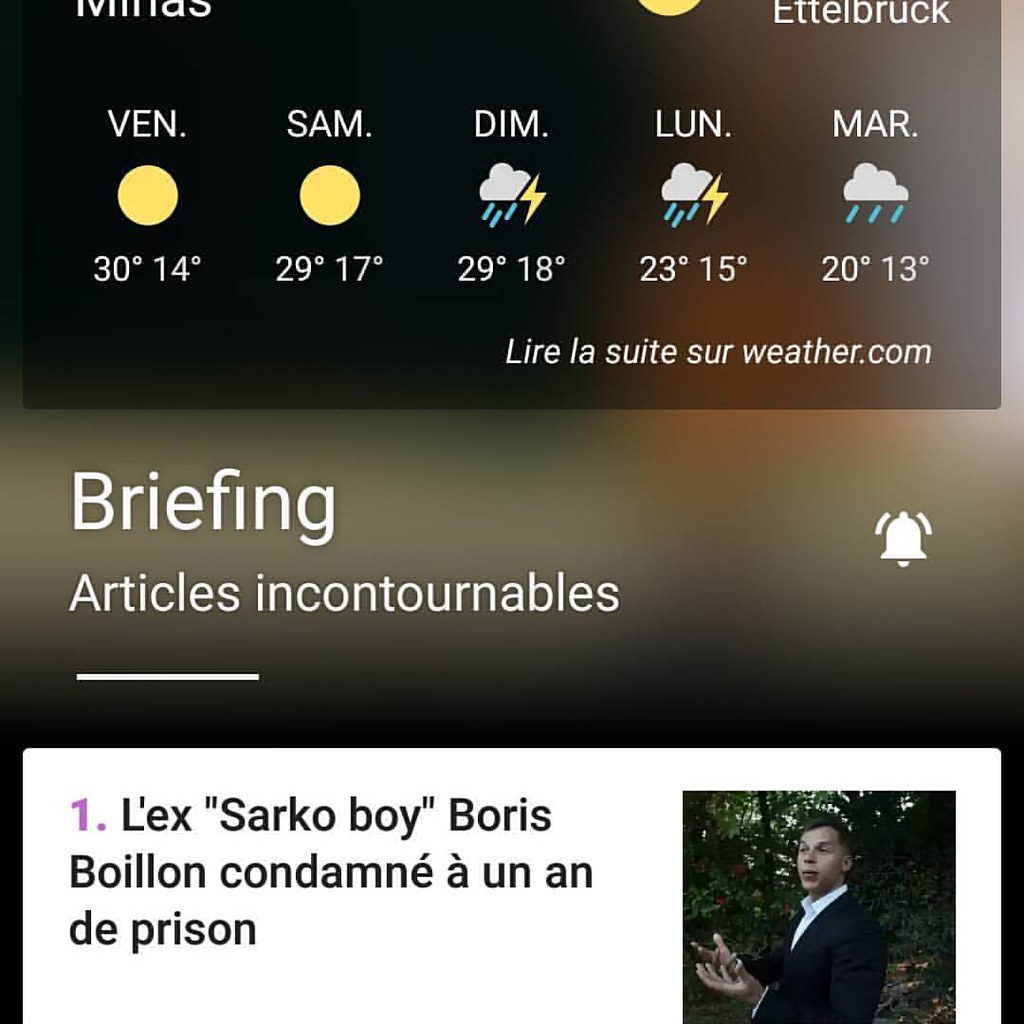This image appears to be a detailed screenshot taken from a mobile device. At the top of the image, there is a black horizontal bar displaying the weather forecast for five days of the week, with the days abbreviated in French. The weather icons include yellow circles indicating sunny days and symbols for thunderstorms and rain, with temperatures displayed in Celsius beneath each icon. In the center of the image, there is a panel labeled "briefing," with the French phrase "articles incontournables" beside it, and a small bell icon on the right. Below this, a white rectangle contains a news story in French: "L'ex-Sarco boy Boris Boyon condamné à un an de prison." This section also features a photograph of a young man, presumably Boris Boyon, dressed in a black suit coat and white shirt, with his hands raised as if gesturing. The text and icons are displayed in various colors including black, white, yellow, light blue, gray, tan, purple, and pink, enhancing the visual engagement of the screenshot. The entire style of the image is characteristic of a mobile device screenshot, designed to be informative and visually structured.